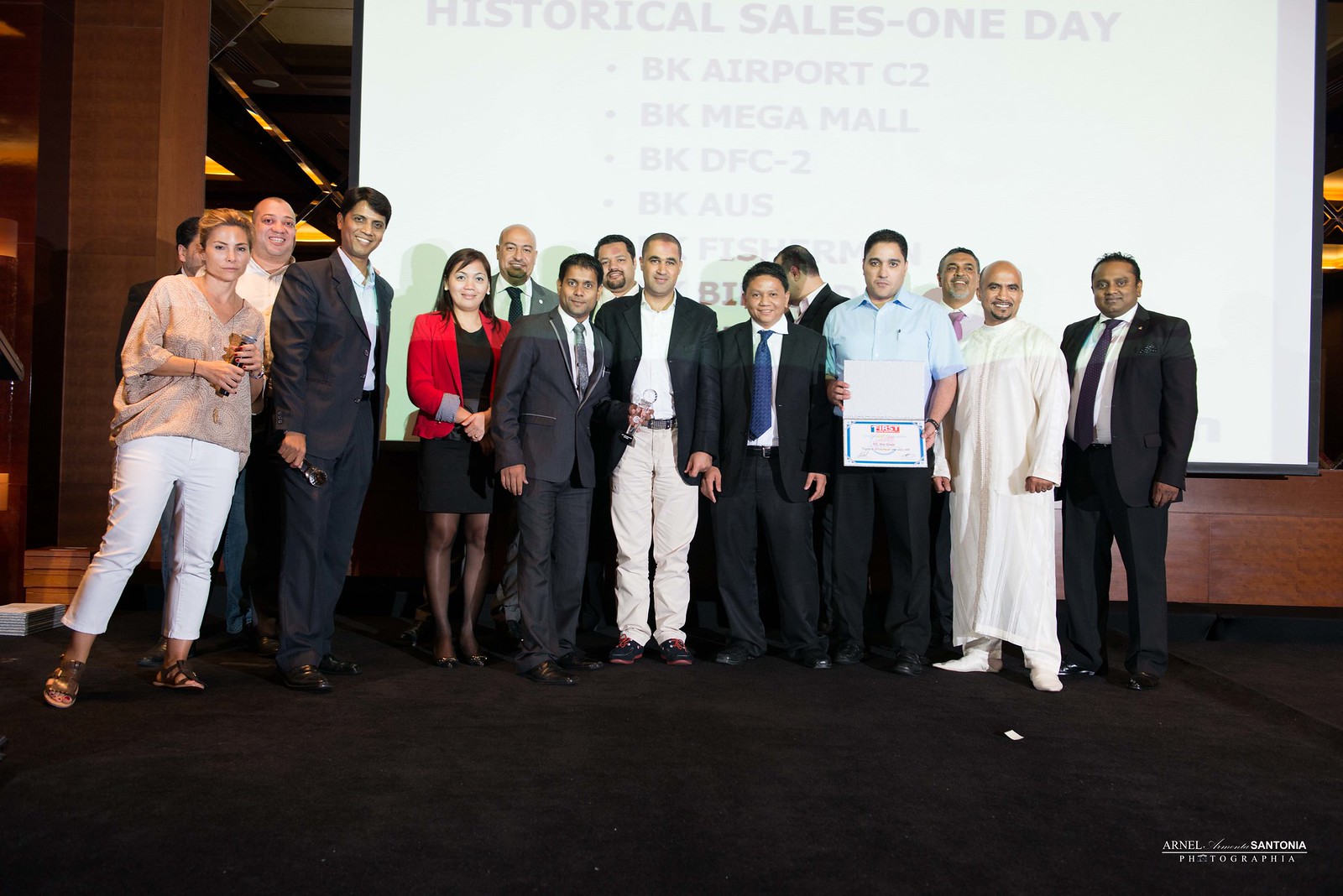The image depicts a group of 14 people standing in front of a large white projection screen with a black border, displaying a presentation slide titled "Historical Sales One Day." The slide lists various locations, including "BK Airport C2," "BK Mega Mall," "BK DFC 2," and "BK Space AUS," with additional bullet points partially obscured by the people. Most of the group is dressed in formal attire, with men wearing suits, ties, and dress shirts in colors such as white, brown, black, and blue. Among them, one individual stands out in a Middle Eastern robe, and another woman is notable for her red blazer paired with a black dress and hose. To the far left, a woman wears white denim capri pants, brown gladiator-style sandals, and a tan blouse. The group appears to be situated in a well-lit, brown-carpeted area, possibly indoors or outside a wood-finished building with a large front window. There is a watermark on the lower right corner bearing the text "Arnell Santonia Photography."